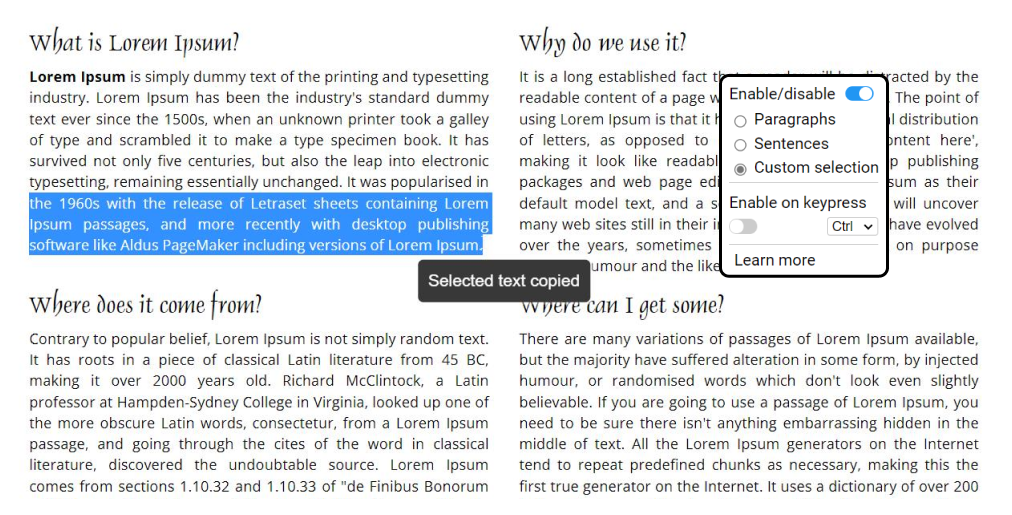In this image, four distinct sections of text are presented against a clean, white background. The text is uniformly black, each section introduced by a bold title. 

The first section, titled "What is Lorem Ipsum?", starts with the phrase "Lorem Ipsum" in bold, followed by a detailed paragraph in regular text. This paragraph describes Lorem Ipsum as dummy text used by the printing and typesetting industry since the 1500s. It explains how an unknown printer created it by scrambling a type specimen book's text. The block has prevailed through centuries and the advent of electronic typesetting, unchanged in essence. Its popularity surged in the 1960s with Letraset sheets and later through desktop publishing software like Aldus Pagemaker. Notably, from "the 1960s" to the end of this paragraph, the text is highlighted in medium blue with white letters.

The second section, titled "Why Do We Use It?", is partially obscured by a small, square-shaped floating toolbox. This toolbox boasts a solid black border and a white interior. It features black text stating "Enable / Disable" and contains three circular buttons labeled "paragraphs," "sentences," and "custom selection." The "custom selection" option has been selected, and its button appears grayed out. Further text in the box reads "Enable on Key Pass," accompanied by a small white and gray dial. Surrounding this dial, on either side, are small boxes marked "CTRL" with downward arrows, and underneath is the phrase "Learn More" in black text. In the upper right-hand corner of the toolbox, a blue-and-white gear icon is activated.

The third section, titled "Where Does It Come From?", reveals that contrary to popular belief, "Warm Ipsum" (likely a typographical error for "Lorem Ipsum") is not random text. It traces its origins to classical Latin literature from 45 BC. The text attributes Richard McClintock, a Latin professor at Hampden-Sydney College in Virginia, with discovering its roots by analyzing the obscure Latin word "consectetur." He identified "Lorem Ipsum" as originating from sections 1.10.32 and 1.10.33 of the work "De Finibus Bonorum et Malorum" by Cicero.

The final section, titled "Where Can I Get Some?", discusses the availability of various "Warm Ipsum" passages. It notes that while many have been altered with humor or random words, genuine passages exist. It warns to ensure the text is free from embarrassing content before use. Online "Warm Ipsum" generators typically recycle pre-defined chunks, making this the first true generator by using a dictionary of over 200 words.

Superimposed centrally on this image is a dark gray rectangle, featuring white text which reads "Selected Text Copied."